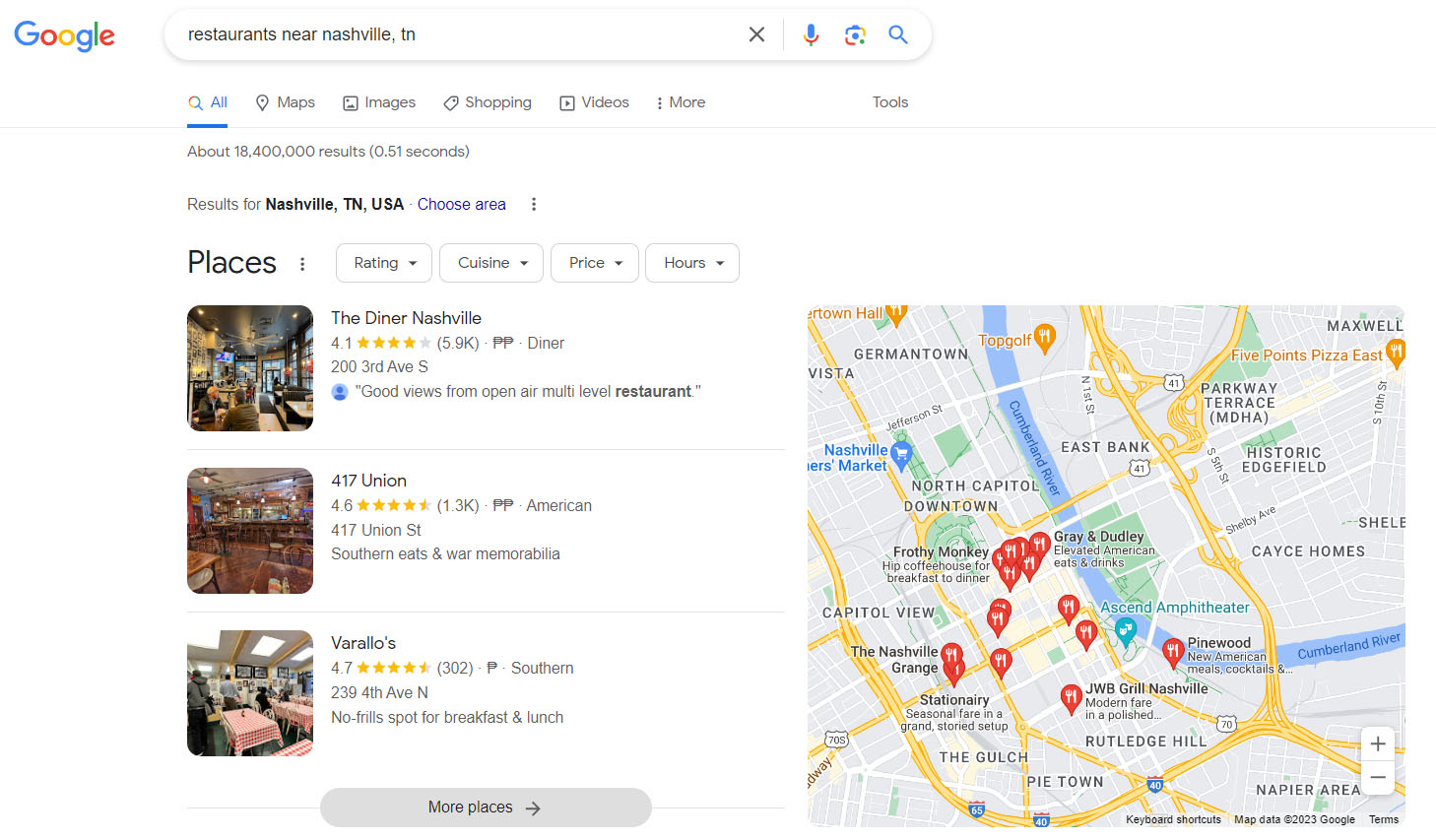Screenshot of a Google search displaying the results for "restaurants near Nashville, TN." In the top left corner, the Google Images logo is visible. Within the search bar, the phrase "restaurants near Nashville, TN" is typed; adjacent to it are icons for canceling the search (a cross), voice search (a microphone), and Google Chrome (an icon), along with the magnifying glass symbolizing the search function. Directly below the search bar, there are category tabs such as All, Maps, Images, Shopping, and Videos, with an additional "More" option for further menu choices.

The search generated approximately 18 million results in 0.51 seconds. The first result appears under a section labeled "Places," showcasing a few featured dining options: The Diner in Nashville, 417 Union, and Varallo's, each accompanied by images of their food and establishment ambiance. A pill-shaped button labeled "More places" is situated beneath this list.

On the right-hand side of the screen, there's an interactive map dotted with pins marked by a knife and fork icon, indicating the precise locations of these restaurants within the Nashville area.